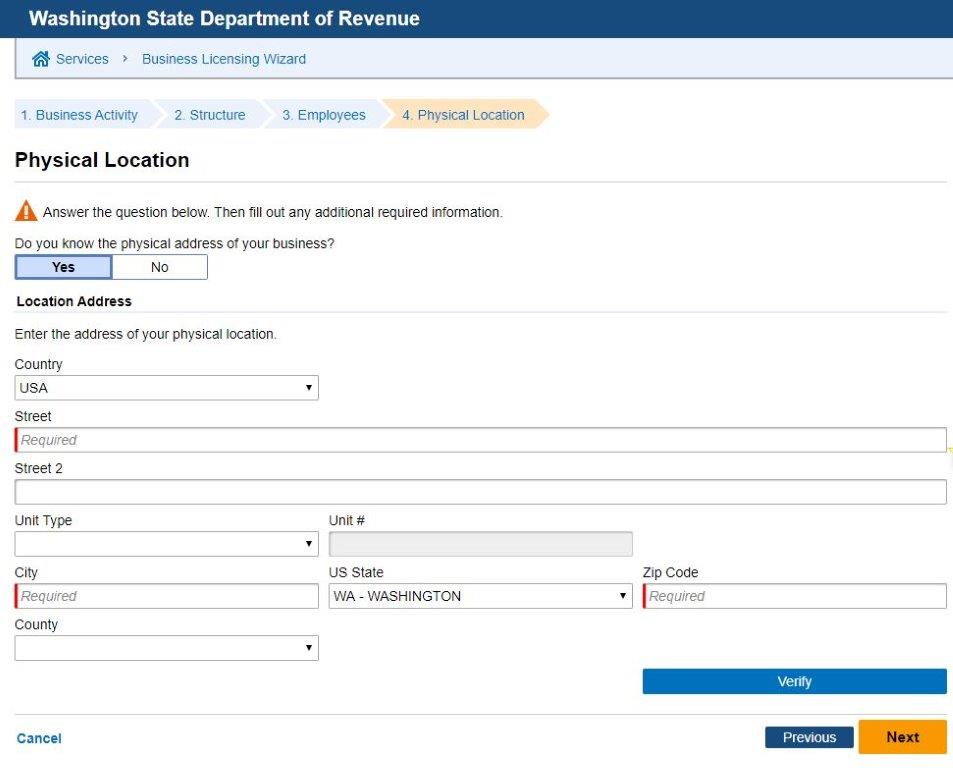This image depicts a webpage from the Washington State Department of Revenue. It appears to be part of their Business License Wizard section.

At the top, the heading "Washington State Department of Revenue" is prominently displayed. Below this, there's a house icon followed by the text "Services". An arrow pointing to the right leads to the "Business License Wizard" section.

The wizard comprises four numbered steps: 
1. Business Activity,
2. Structure,
3. Employees,
4. Physical Location.

Currently, the "Physical Location" step is active, highlighted in bold black text. Beneath this, a caution symbol is displayed alongside the instruction: "Answer the questions below, then fill out any additional required information."

The webpage is asking if the user knows the physical address of their business, presenting two buttons labeled "Yes" and "No". The "Yes" button is highlighted in blue.

Further down, the form solicits the location address details:
- "Country" is pre-filled with "USA", accompanied by a drop-down arrow.
- "Street 1" is marked as a required field.
- "Street 2" is an optional field.
- A drop-down menu for "Unit Type" is available but unfilled.
- An empty "Unit Number" field in grey.
- "City" is required.
- "State" is pre-selected as "WA - Washington".
- "ZIP Code" is a required field.
- "County" is at the bottom, with a drop-down arrow for selection.

Finally, at the bottom of the form, there are blue "Verify" buttons, along with "Previous" and "Next" navigation buttons, allowing the user to move through the steps.